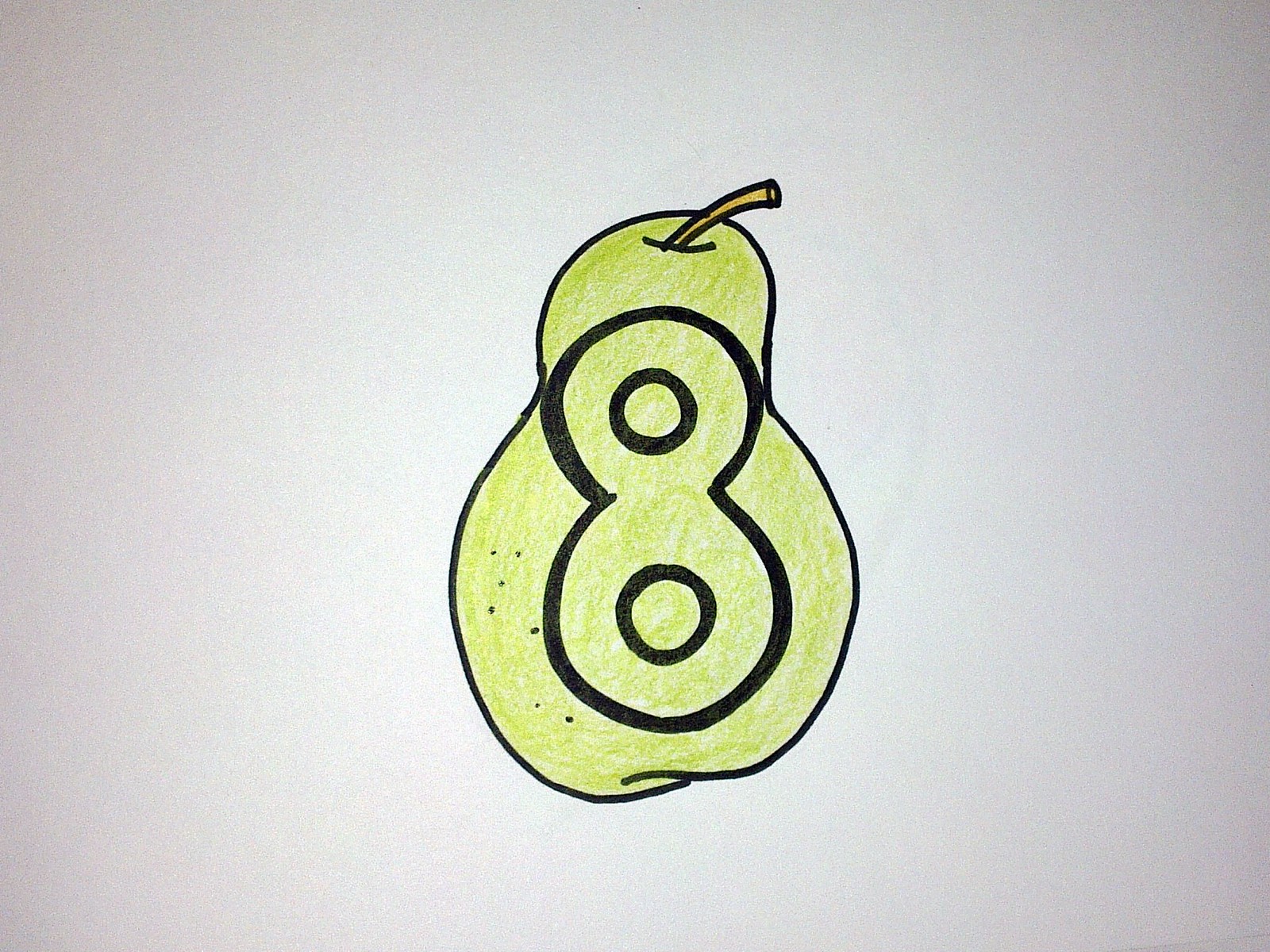The image depicts a hand-drawn illustration on a piece of white paper. The centerpiece is a pear, outlined in black marker and colored in green. The pear has a light brown, cylindrical stem that tilts sideways. The bottom of the pear features an overlapping line to mimic the natural indentation found in real pears. At the core of the pear, taking up its entire length, is a large, chunky numeral eight, also outlined in black marker. This number has an H-like shape with equally sized top and bottom sections, giving it a three-dimensional appearance. The image has subtle black dots on one side of the pear, enhancing its detailed, albeit amateurish, look. The background of the drawing is white, but there is a gray tint, creating an effect of light that is brighter in the middle and darker towards the edges.